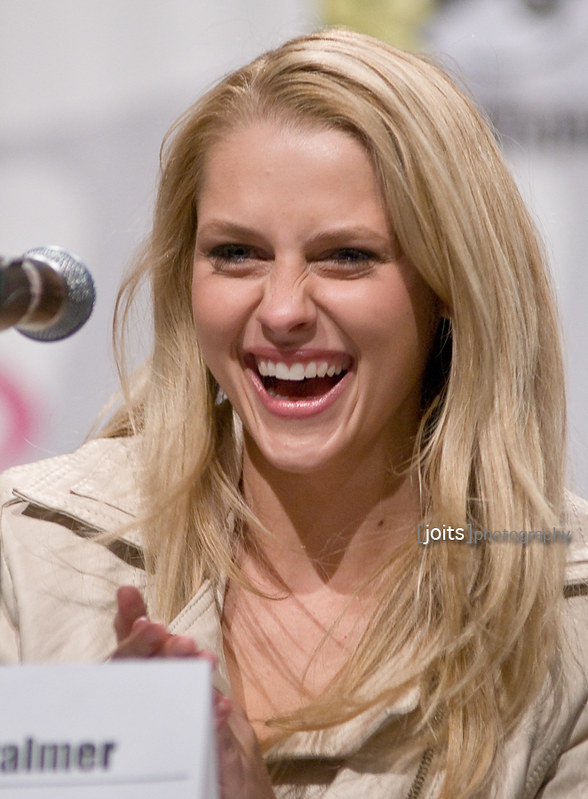In this vertically aligned rectangular photo, a woman with layered blonde hair that cascades past her shoulders is prominently featured. She has white skin and blondish-brown eyebrows. Her smile is broad, showing her teeth, and her eyes are squinted with laughter. Her hands, appearing to clap their fingertips together, are visible in front of her. She is wearing a beige or tan-colored zip-up jacket or collared shirt, and the image is cropped to show her from the chest up.

To her right within the frame, the words "JOINTS Photography" are visible, with "JOINTS" in white letters and "Photography" in gray letters. In the upper left-hand side of the photo, the silver tip of a microphone can be seen. Additionally, a sign reading "A-L-M-E-R" in black letters is partially visible in the lower left corner. The background is a blur of white and gray tones, adding to the focus on the smiling woman, who may be an actress.